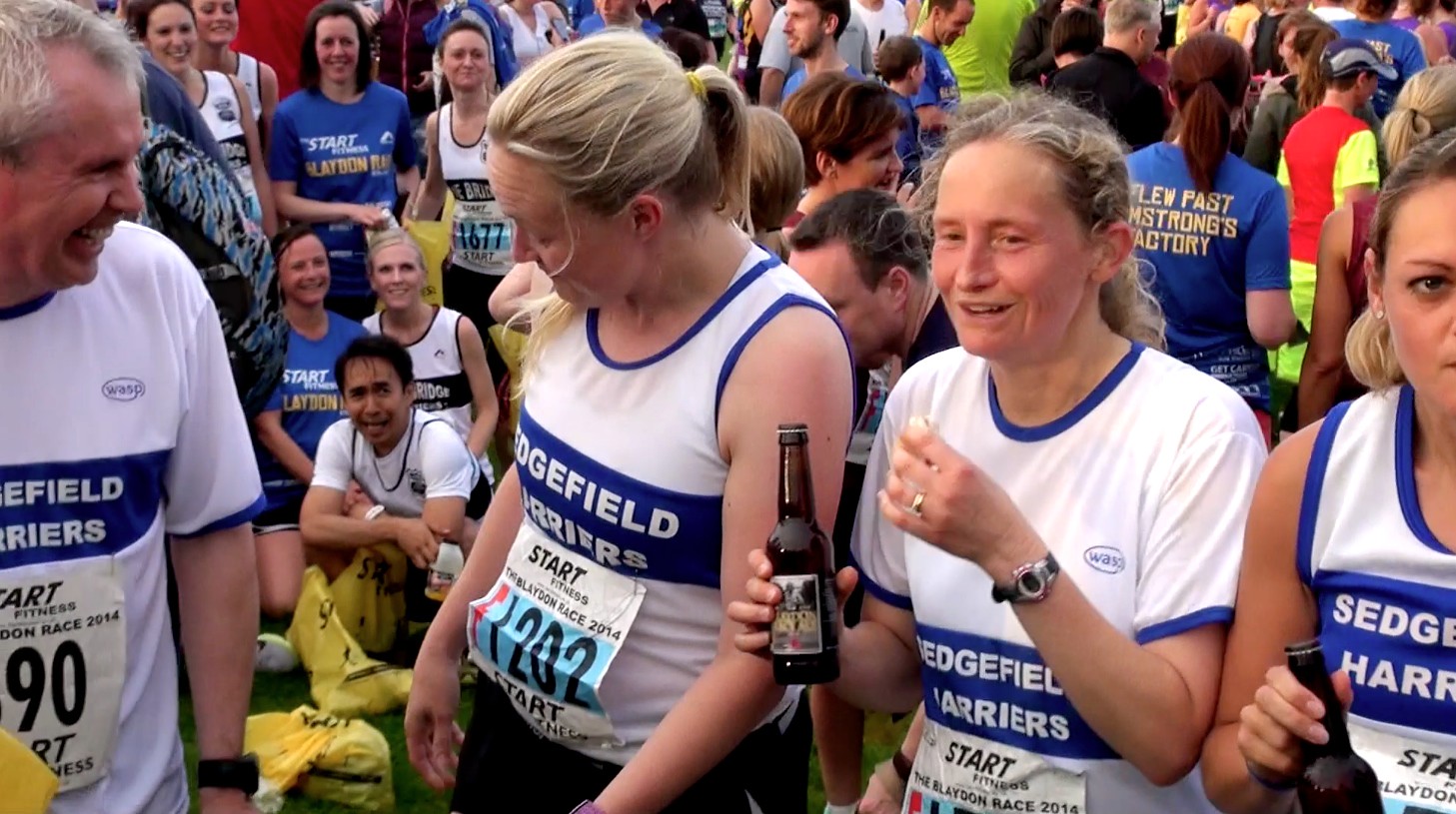This horizontally aligned rectangular photo captures the aftermath of what appears to be the Bladen Race in 2014, organized by the Sedgefield Harriers. In the foreground, there are four main figures—a mix of three women and one man, all wearing matching athletic shirts featuring a white and blue design with the 'Sedgefield Harriers' logo. The shirts vary slightly, with some being short-sleeved and others tank tops. Each has race numbers pinned to their waists: the woman in the tank top has the number 1202, while the man’s number partially appears as 90, though it might have digits preceding it. The woman on the far right, who has blonde hair pulled back and is wearing stud earrings, is gazing directly at the camera; however, she is only partially visible due to the photo’s framing. Both she and another woman next to her are cheerfully holding beverages that resemble beer bottles, highlighting a celebratory mood. The lively background features a crowd of supporters and fellow racers, some turning towards the camera and others facing away, contributing to the festive atmosphere. People in blue shirts apart from the athletes seem to be event staff or volunteers, reinforcing the communal spirit of the event.